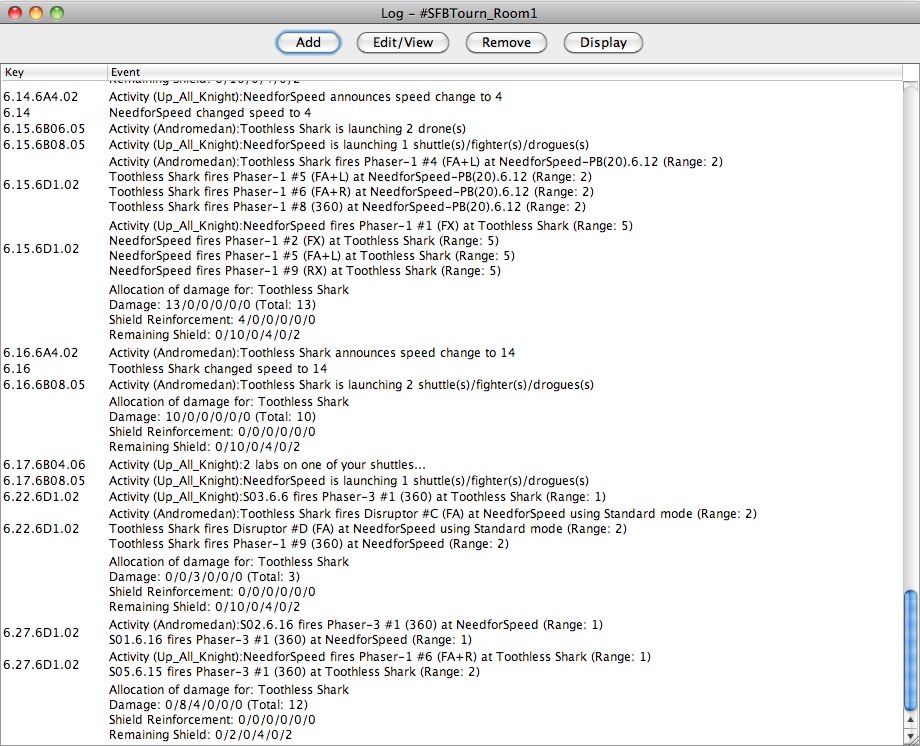The image showcases a detailed computer interface with a long log displayed on an all-white background. 

In the upper left corner, there are three circular buttons in red, yellow, and green. Below these buttons, a gray-shaded header displays the text "Log SFBTOURN_Room 1." Beneath the header, five operation options are clearly visible: Add, Edit, View, Remove, and Display, each accompanied by its own circular white button.

The log consists of multiple columns, with key details and events prominently featured. The key contains various numbers, each corresponding to different activities recorded in the log. The event column includes descriptions of activities, such as "Toothless Shark is launching" or details about "Need for Speed range" and the allocation of damage for each section.

All the text is presented in black font on a pristine white background, ensuring clarity. Notably, the log does not include any specific dates or times, focusing solely on the activities and their descriptions. Along the right edge of the interface, there is a blue scroll button, facilitating navigation through the extensive log.